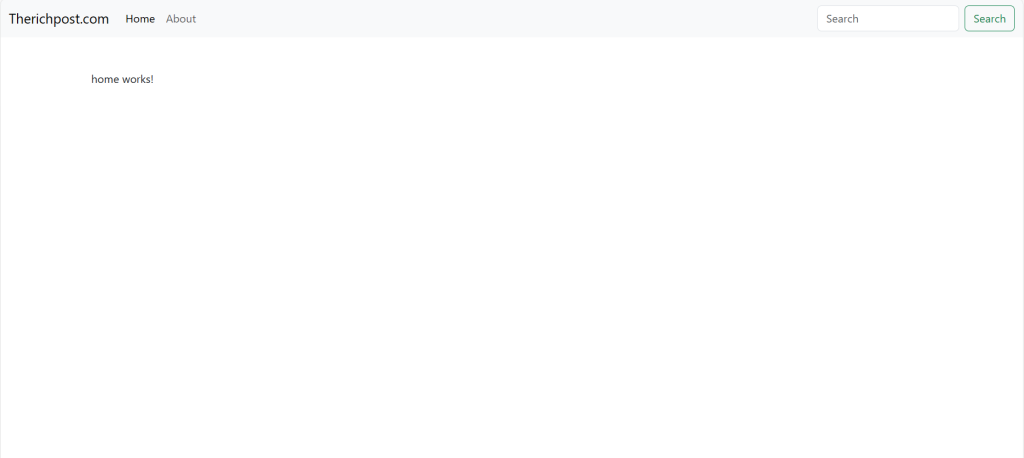The image depicts a predominantly blank screen with minimal elements visible. At the top of the screen, there is a faint blue stripe that features the text "therichpost.com" in all lowercase letters, except for a capital "T." This stripe also includes menu items such as "Home" and "About," with "About" appearing faint. Towards the right end of this stripe is a search bar containing the placeholder text "search," which is also faint, but the word "search" next to it is highlighted in blue.

Directly below this stripe, in the center of the otherwise blank space, the words "homeworks!" appear in all lowercase letters and a gray font, though it is not bold. The text "therichpost.com" and "homeworks!" stand out slightly more against the sparse background due to their bolder appearance compared to the other faint elements.